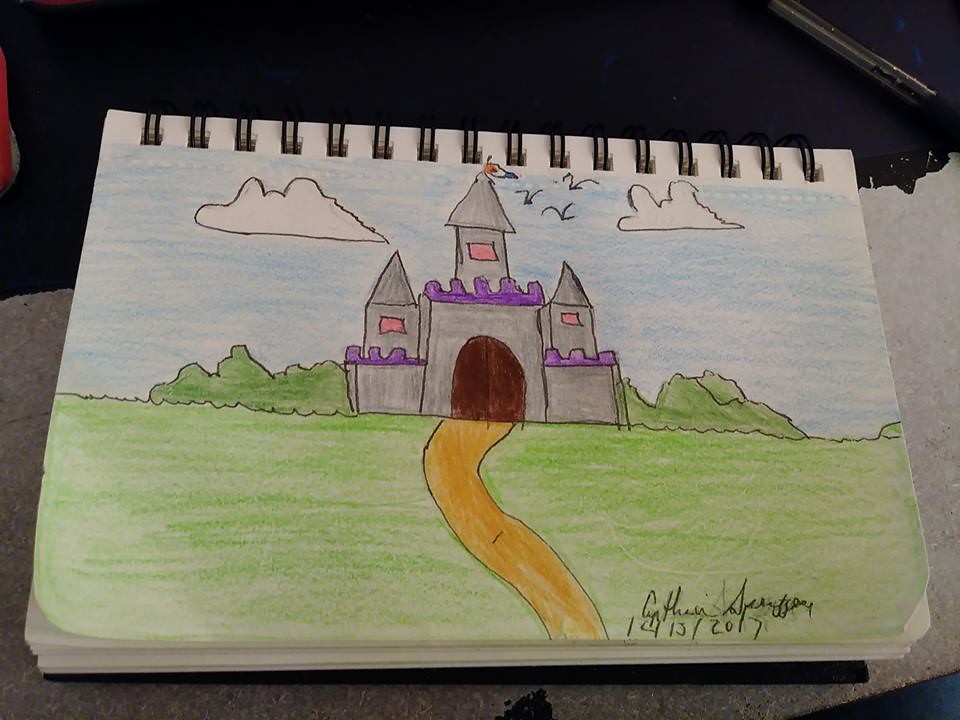This photograph captures a colorful crayon drawing in a spiral-bound notebook, showcasing a whimsical castle. The stone-colored structure features three towers—the tallest one in the center flanked by two shorter ones, each adorned with vibrant purple turrets. The castle’s pink windows and a sturdy brown wooden door add charming details to the scene. A light, curved dirt path extends from the door to the foreground, bordered by lush green grass. Shrubs flank the castle on either side, enhancing its fairy-tale allure. Above, a serene blue sky is punctuated by two clouds—a large one on the left and a smaller one on the right. Near the towering center spire, three bird silhouettes soar, adding a touch of life to the scene. At the pinnacle of the tall central tower, a red, white, and blue flag flutters in the breeze. The drawing is signed in the bottom right corner with "Cynthia S—" and dated "12/13/20," indicating the artist and the creation date. The playful and vibrant crayon texture suggests a youthful creator, adding to the drawing's enchanting charm.